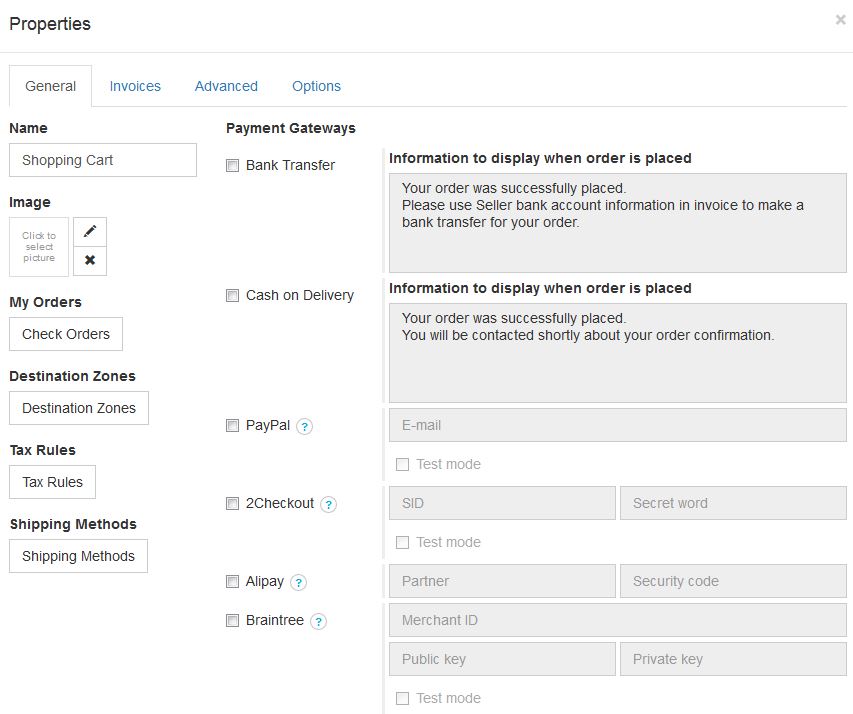A screenshot is displayed showcasing a software interface with various tabs and options. At the top, there are five main tabs: "Properties," "General," "Invoices," "Advance," and "Options." The "General" tab is highlighted in gray with a rectangular border around it, indicating it is currently selected, while the other tabs are blue, signifying they are not active.

Within the "General" tab, there are fields labeled "Name" and "Shopping Cart," where users are likely meant to input details for the current item or service. Additionally, there's a section entitled "Information," specifying details to display when an order is placed. 

On the left-hand side of the interface, there are several headings with accompanying editable boxes. These include:
- "Image": A box beneath it prompts users to "Click to select picture."
- "My Orders": Below this, a box with the option to check orders.
- "Destination Zones": Followed by a box related to the respective destination zones.
- "Tax Rules": Underneath is a box for inputting tax rule details.
- "Shipping Methods": With a box under it for selecting shipping methods.

To the right side of the interface, under "Payment Gateways," several payment options are listed, including "Bank Transfer," "Cash on Delivery," "PayPal," "2Checkout," "Alipay," and "Braintree," allowing users to configure their preferred payment methods.

Overall, the design appears to be an administrative panel section of an e-commerce platform, enabling users to configure various settings related to orders and transactions.